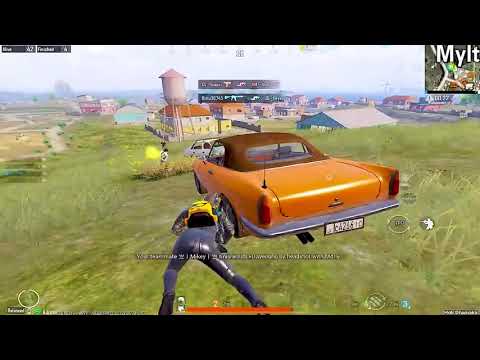The image is a widescreen screenshot from a video game that strongly resembles Fortnite. It features dramatic black bars at the top and bottom, with various in-game elements overlaid. The upper right-hand corner contains the partially obscured text "MYLT" in white font with a black border, alongside a mini-map and possible machine gun and score icons.

Central to the image, an orange vintage car with a brown ragtop roof is prominently positioned slightly angled, as if facing to the left. In front of this car, a character wearing shiny black leather pants and a yellow backpack is crouched, seemingly taking cover. To the character's left in the distance, another person is visible, potentially engaged in a firefight, with evident gunfire.

The scene takes place in a grassy field on a hill, with a background showcasing a small town. Notable structures include a gray water tower, a large blue building with a tin roof, and buildings with prominent orange roofs, all under a somewhat cloudy horizon. The overall quality of the image appears low-resolution, showing signs of compression. Finally, there are rectangles with text at the top and a red stripe at the bottom, possibly indicating health or game progress metrics.